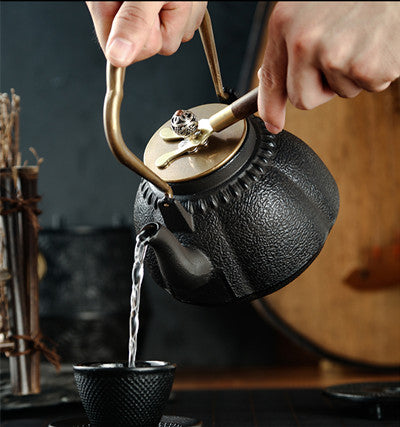In this professionally staged and meticulously lit photograph, we see a detailed black cast iron teapot with a brass handle and a lid, characterized by its garlic-shaped body with little rounded lobes. The teapot is pouring hot water into a black cup. One hand holds the handle of the teapot while the other uses a brass-ended tool to secure the lid as the water is poured. The background is softly out of focus, subtly revealing cinnamon sticks wrapped into a vertical column and what appears to be another pot, along with a few indeterminate wooden objects that could be instruments or decorative items. The setting suggests a comforting scene, possibly in a home or a restaurant, highlighting the intimate moment of preparing a hot beverage, most likely tea.